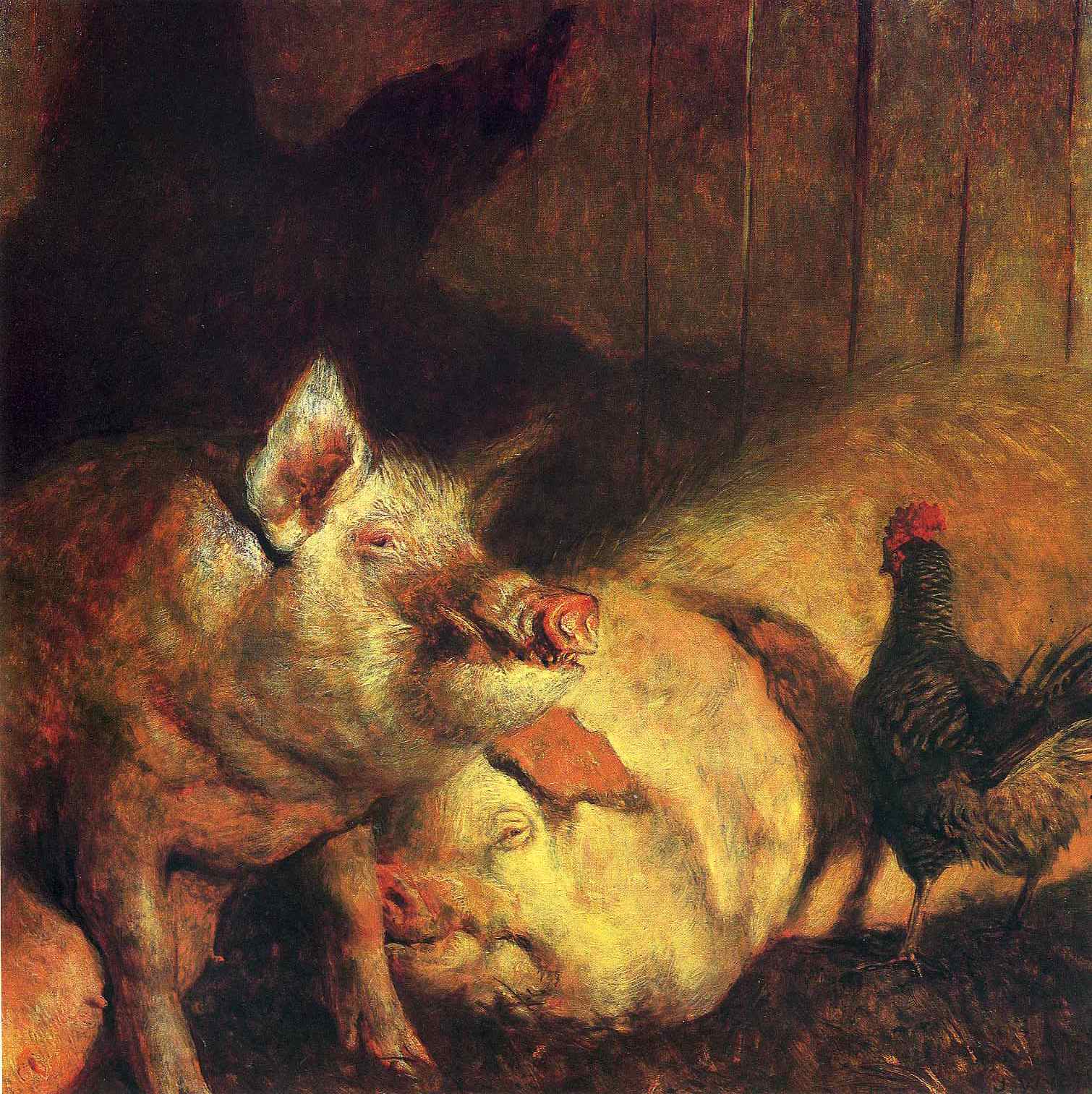This painting depicts the interior of a barnyard with a close-up view of three animals. Dominating the scene on the left is an upright warthog or pig, sitting on its hind legs with its front legs up, its gaze directed forward, and its teeth partially visible. To the left of this warthog lies a massive, fat pig sprawled on the ground, appearing half-asleep with its eyes open. Its positioning and the surrounding hay suggest a serene, yet somewhat weary demeanor. Positioned to the right side of this large pig's head, slightly turned away from us and facing the resting pig, is a rooster with distinctive red feathers atop its head. The rooster stands with its back to the viewer, adding a silent, observational presence to the tableau. The detailed brushwork blends the barn’s earthy tones, creating a cozy yet rustic atmosphere that envelops the entire square-framed scene.